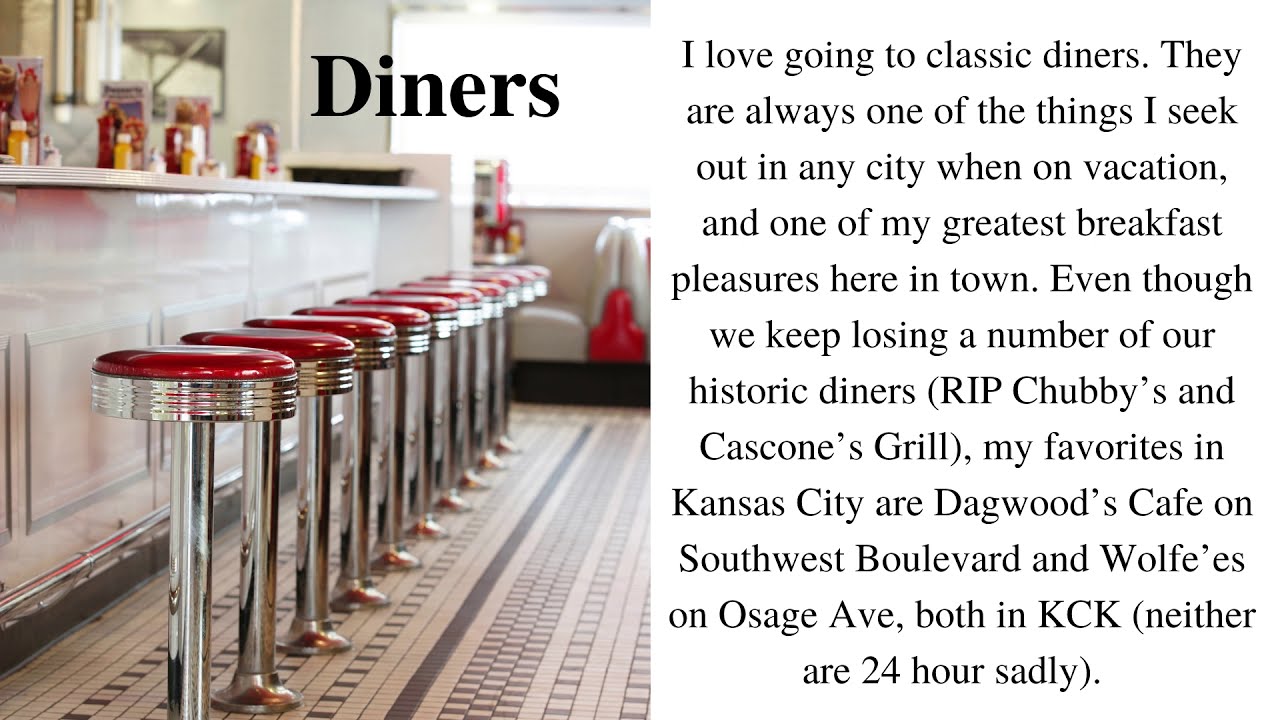In the left half of this graphic, there's a nostalgic photograph capturing the essence of a classic diner, reminiscent of the 1940s and 1950s. The image is taken from knee level, showcasing a row of vintage diner stools. The stools feature shiny, bright red vinyl seats perched atop chrome and ribbed posts that are bolted to the floor. In front of the stools, there is a slick, white counter adorned with a neat row of condiment bottles, including red ketchup, yellow mustard, salt, and pepper. A small brochure, likely the menu, is also visible among the bottles. Further into the background, red and white booths add to the authentic diner ambiance. Overlaying the photograph in black, bold Times New Roman font, the word "diners" is prominently displayed.

The right side of the graphic contains a heartfelt paragraph in black text: "I love going to classic diners. They are always one of the things I seek out in any city when on vacation and one of my greatest breakfast pleasures here in town. Even though we keep losing a number of our historic diners, rest in peace Chubby's and Cascone's Grill. My favorites in Kansas City are Dagwood's Cafe on Southwest Boulevard and Wolf's on Osage Avenue, both in KCK. Neither are 24 hours, sadly."